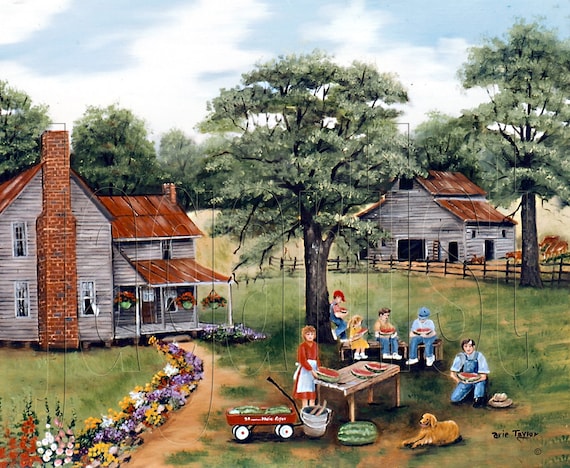This detailed painting depicts a serene and vintage farm scene brimming with familial charm. On the left side stands a white farmhouse with a distinctive red brick chimney climbing its front façade and topped by a bright red roof. Adjacent to the farmhouse, a picturesque walkway lined with hanging plants and flowerbeds leads to its welcoming porch. Dominating the background to the right, a matching white barn with a red roof and surrounded by a fence marks the boundary of this pastoral setting. Just in front of the barn, a tall tree with vibrant green leaves provides a backdrop to the scene.

In the heart of the painting, a second towering tree stands as a centerpiece where a family enjoys a small but joyous picnic. Beneath its shade, a mother, dressed in a long-sleeved dress with an apron, stands by a table laden with freshly cut watermelon pieces and another whole watermelon resting on the ground nearby. She has a bucket ready for the rinds. To her side is a red flyer wagon filled with more watermelons. The father, donning his bib overalls, sits on the grass to the right, savoring a sweet slice of watermelon with his hat placed beside him. Near him, a light brown dog, possibly a golden retriever, relaxes on the ground.

Further into the foreground and extending towards the barn, four children are indulging in the juicy fruit. Three of them—two boys and a girl in a yellow dress—are seated on a bench, while a fourth boy leans nonchalantly against the tree with his foot propped up, wearing a red cap and enjoying his watermelon. In the distance, meadows and possibly some livestock enhance the rural essence of the painting, which is delicately signed "Aerie Taylor" in the lower right corner. This artwork captures a moment of pure, idyllic bliss in the countryside.